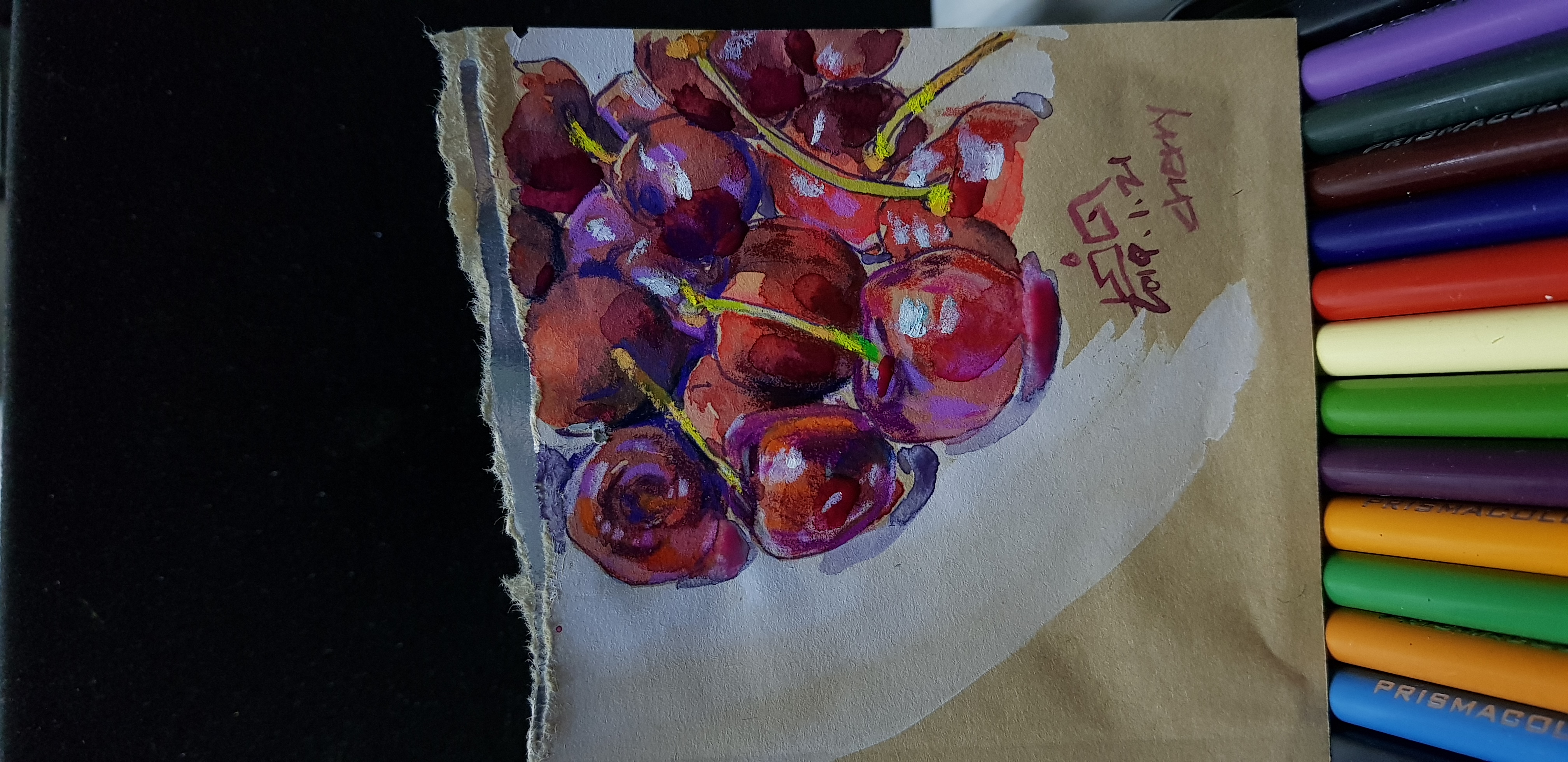The image is a detailed drawing of vibrant, juicy red cherries with light green stems, depicted on a piece of white paper that appears torn at the top. The cherries are skillfully rendered, with white reflection spots that make them look wet and three-dimensional. Purple is used as an accent color, both on the cherries and in the shadowing beneath them, adding an otherworldly feel. To the right side of the image, there is a set of colored pencils, likely used for the drawing. The pencils are arranged in an orderly fashion and come in a variety of colors: purple, dark purple, blue, dark blue, teal, green, forest green, brown, yellow, orange, white, and red. Some pencils bear the text "PRISM." The left side of the image shows a black void. The drawing, possibly on a brown and white bag-like material, features more than a dozen cherries of varying sizes. The bottom right corner of the image includes the date "2019.1.21" with the word "cherry" written in red text below it.